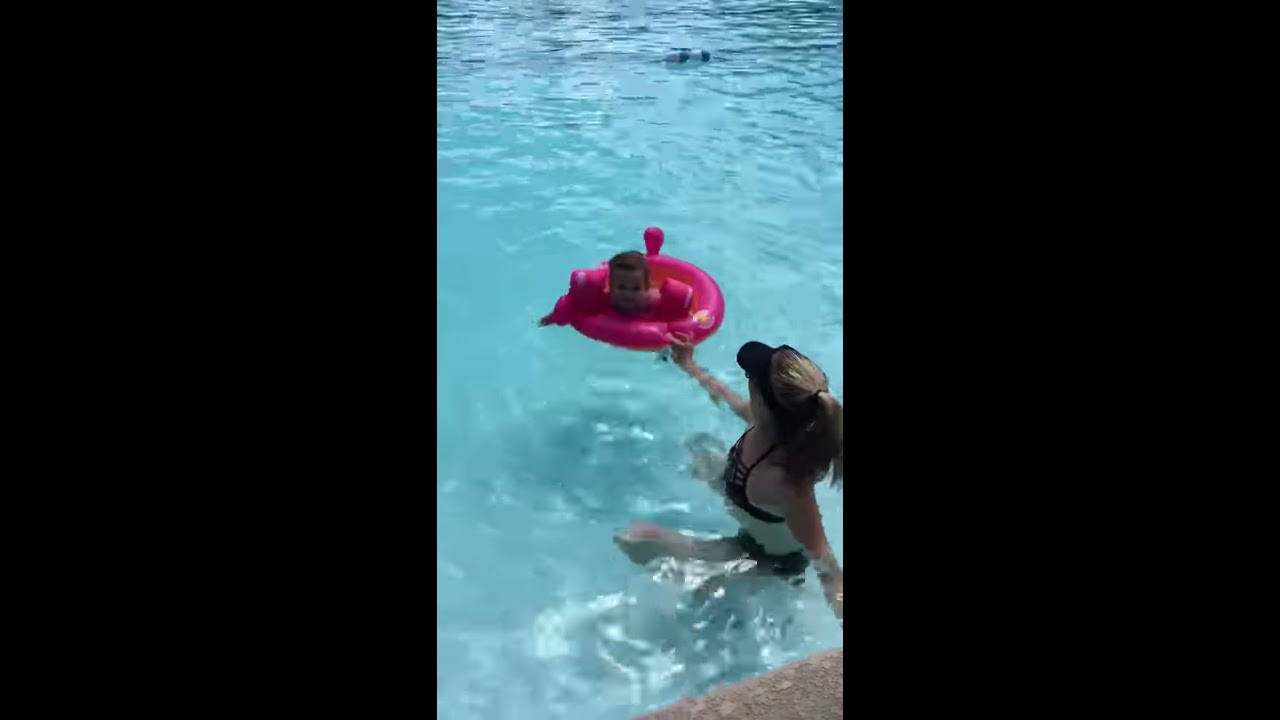In the image, a young child with tan skin and short black hair is floating in a clear, light blue swimming pool. He is surrounded by a dark reddish-pink circular float and wears matching shoulder floats. The child is paddling slightly and looking up and to the left, his face partially visible. A woman, with her hair in a dark brown ponytail and wearing a black one-piece swimsuit with a white waist area, is holding onto the float with her right hand while grabbing the edge of the pool with her left hand. Most of her lower body is submerged in the water, while her upper body remains above the surface. The scene is framed vertically with black borders on the left and right sides, and the water glistens with reflections of sunlight. The stone edge of the pool is visible in the lower right corner of the image.